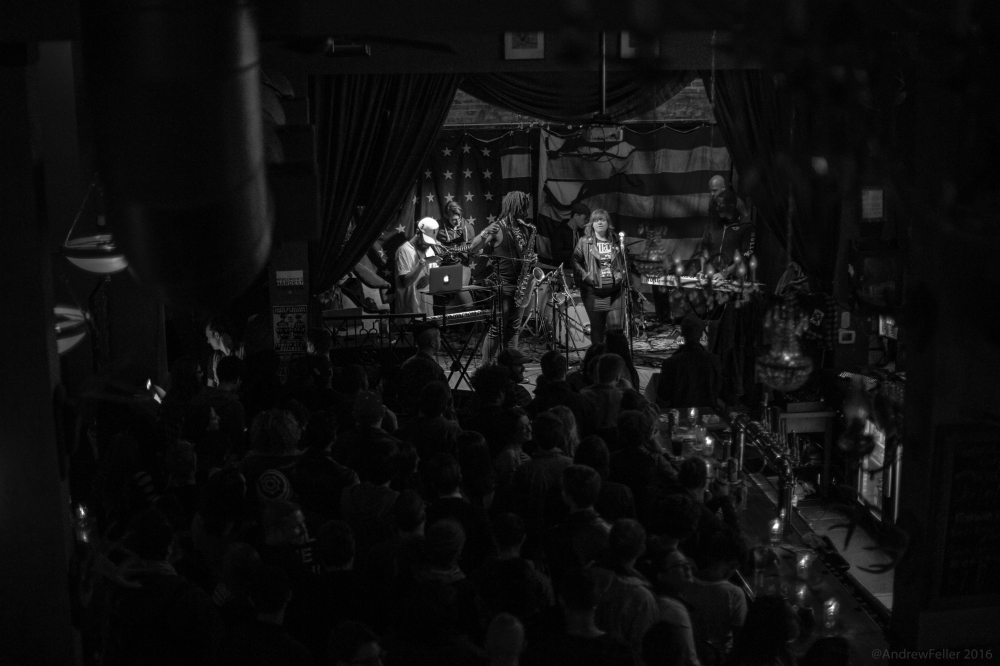This black and white photograph captures a dimly lit scene of a live musical performance, likely taking place in a club or bar. The stage is framed by a dark backdrop featuring fabric with what may be a stylized American flag theme—stripes on one side and stars on the other. In the center, a curtain is draped from both sides, swooping down slightly.

Three to six performers are visible on the stage. To the left, a man in a dark vest and pants is playing a saxophone or tuba, while another person, potentially a woman in a jacket and graphic tee, is positioned next to him at a microphone. Further in the background, a man in a white t-shirt and hat is stationed behind an Apple-logoed laptop. Another performer seems to be playing a keyboard. The scene suggests a small intimate venue with low, moody lighting, which only allows the dark outlines of the audience's heads to be visible in the foreground. Overall, the photograph encapsulates the atmosphere of a lively yet shadowed concert setting.